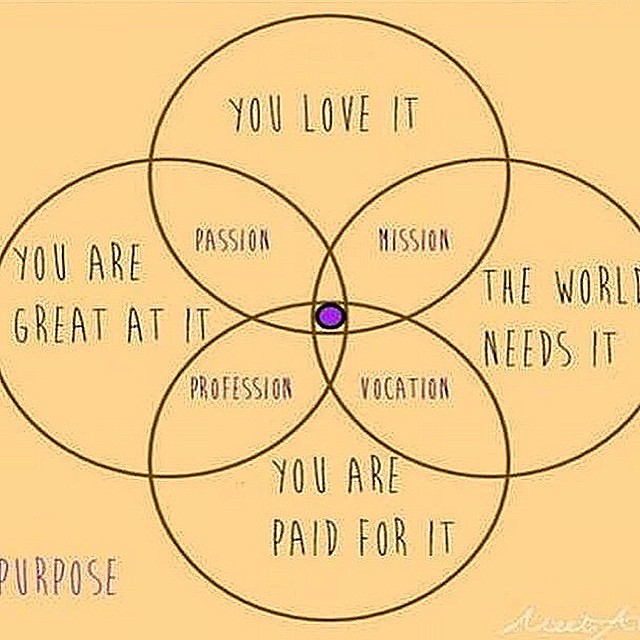The image is a detailed and colorful Venn diagram comprising four interlocking black circles with handwritten text, all set against a peach or yellow background. The top circle is labeled "You love it," the right circle "The world needs it," the bottom circle "You are paid for it," and the left circle "You are great at it." At the intersections of these circles: the top and left overlap to form "Passion," the left and bottom overlap to form "Profession," the bottom and right overlap to form "Vocation," and the top and right overlap to form "Mission." At the very center, where all four circles intersect, there is a smaller purple circle outlined in black that denotes "Purpose," representing the convergence of these elements. Additionally, there is an illegible white cursive signature at the bottom right of the image.